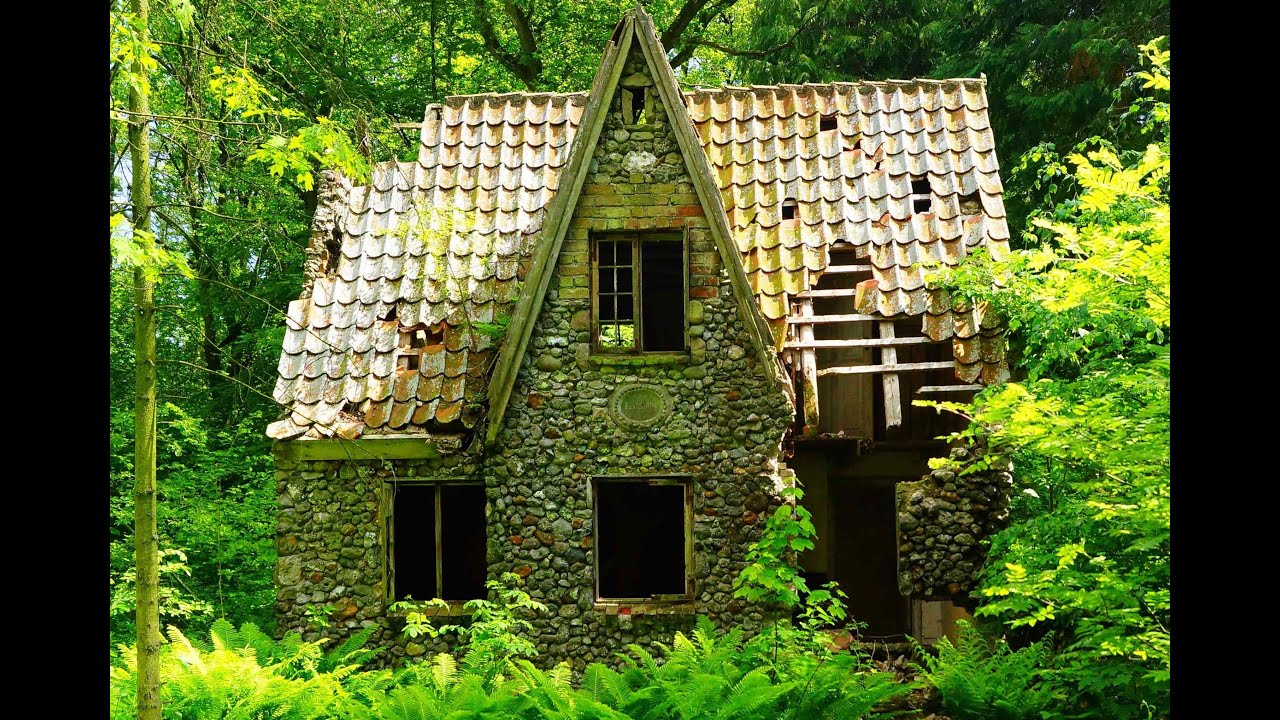The image depicts an old, abandoned cottage nestled in a lush, green environment with ferns, tall trees, and dense shrubbery. The front view, captured in color, shows a cottage in severe disrepair, characterized by its distinct sharply angled, peaked roof. The roof, originally made of wooden or terracotta shingles, now has many missing or broken shingles, particularly on the right-hand side where the internal structure is exposed. 

The walls of the cottage are predominantly constructed from cemented river stones, with some brickwork around the windows. A notable feature is a stone plaque situated between the front door and a second-floor window, likely intended for a name inscription. All the windows are broken, and the overall state of the cottage—a mix of missing shingles, broken windows, and structural gaps—suggests it has been abandoned for many years. The overgrown vegetation further emphasizes the long period of neglect, giving the structure a haunted, forgotten appearance amidst the forest greenery.